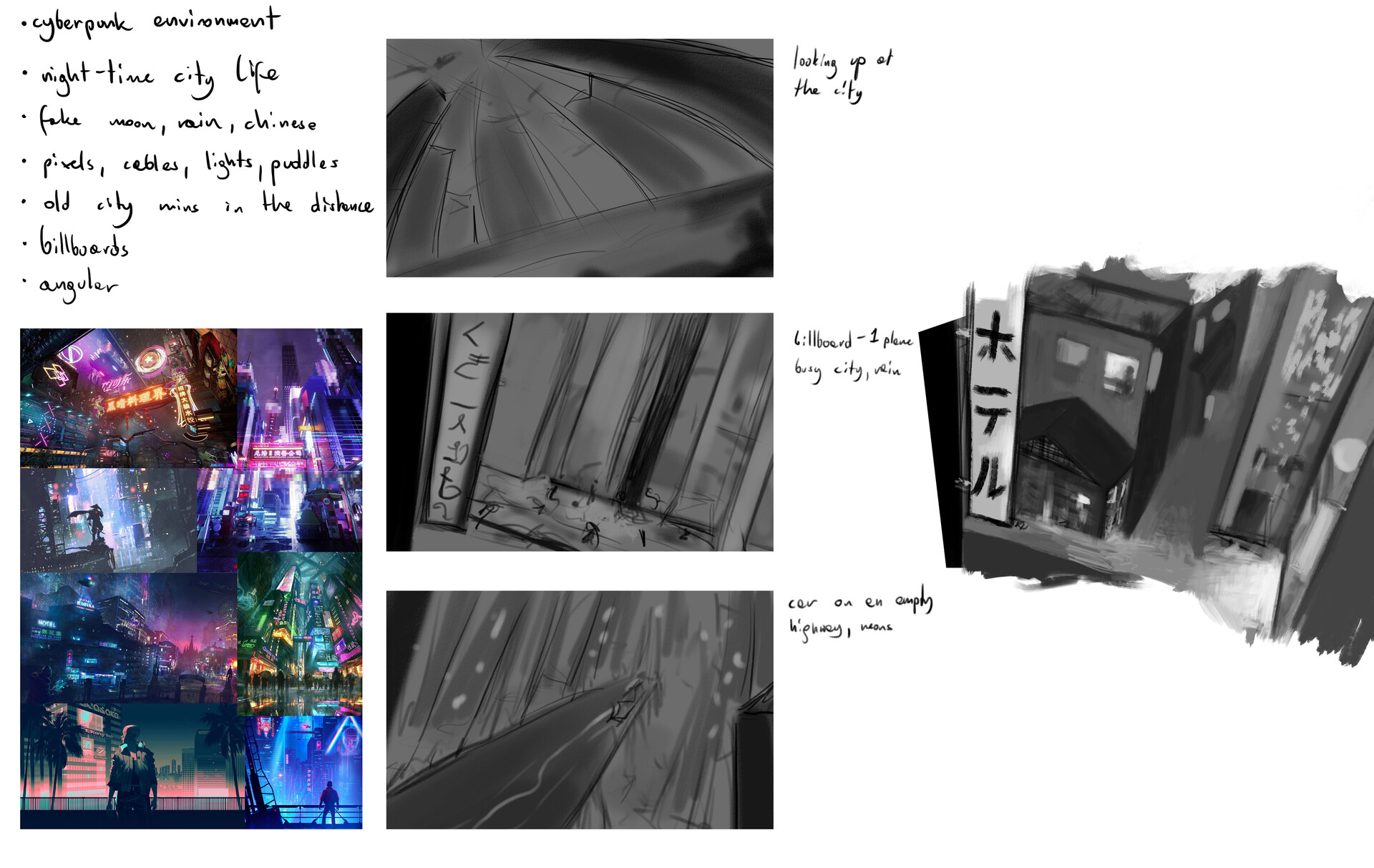The image is a storyboard comprising five different frames, primarily in black and white, with one vividly colored panel. The upper left features a detailed bullet-point list describing a "cyberpunk environment," including elements like "nighttime city life," "fake moon," "rain," "Chinese characters," "pixels," "cables," "lights," "puddles," "old city elements in the distance," and "billboards." The colored panel, located at the bottom left, is rich in neon hues such as purple, blue, orange, and pink, adding a vibrant contrast to the monochromatic scheme of the other frames. The scenes depicted evoke a futuristic, dystopian atmosphere reminiscent of "Blade Runner," showcasing a busy city with digital billboards, rain-soaked streets, and angular architecture. Text labels within the frames include phrases like "looking up at the city," "billboard," "busy city," and an illegible small black writing at the bottom. The overall composition suggests a cinematic vision of a bustling cyberpunk metropolis, filled with intricate urban details and dynamic lighting.